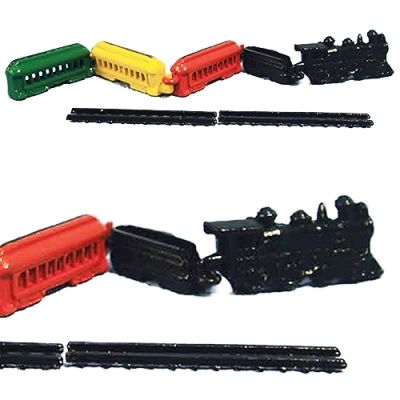The image features two photographs of a colorful toy train arranged one above the other. The top photograph captures the entire model train: a black steam engine followed by a black coal car, then three passenger cars in red, yellow, and green. Set on simple black tracks, two detached pieces of track lie in the foreground. The lower photo is a zoomed-in version, focusing closely on the steam engine, the coal car, and part of the red passenger car, offering a closer view of the simplistic details of the plastic toy. Both images highlight the train’s minimalistic design and colors, set against the unobtrusive black tracks.